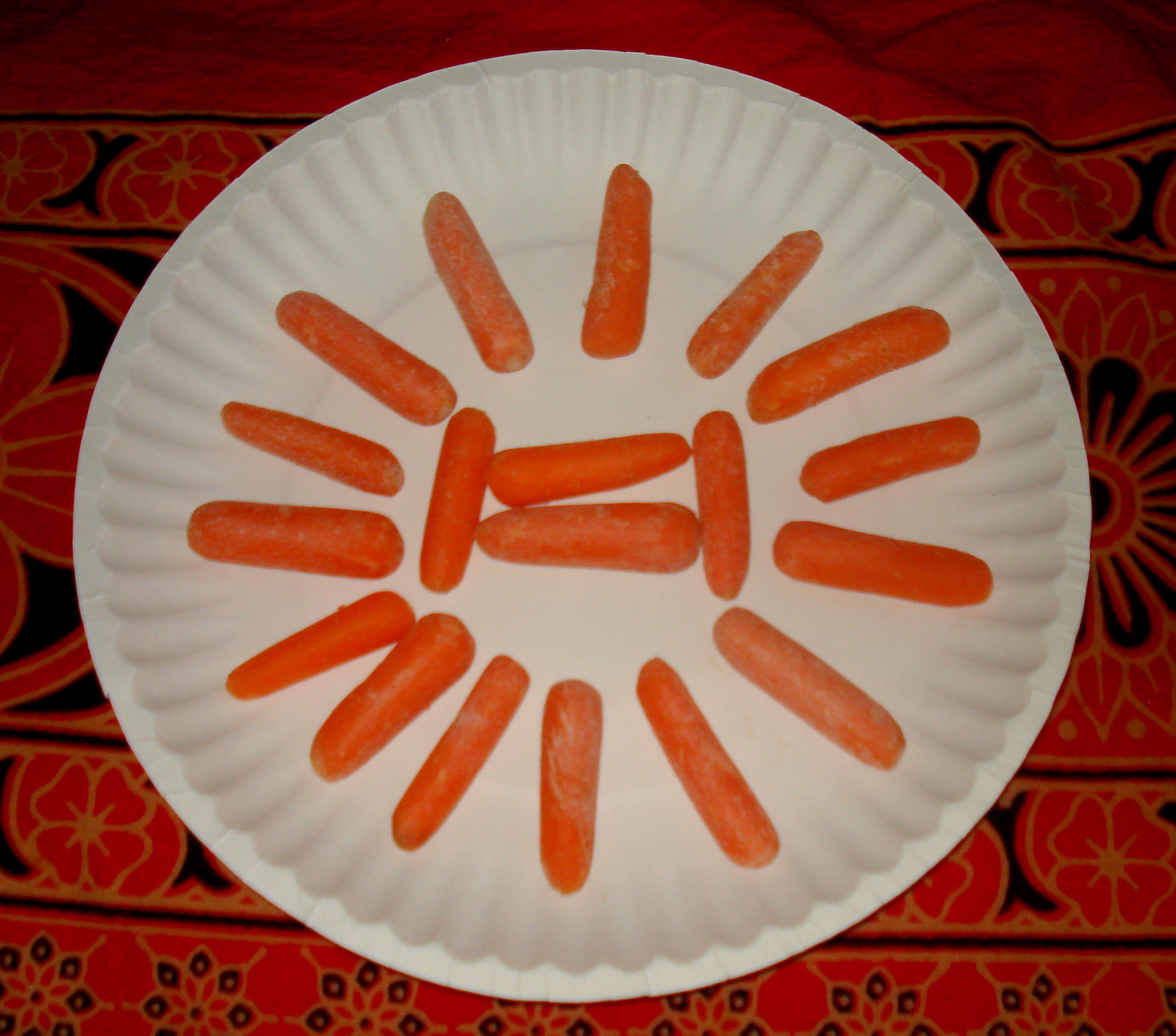This photograph features a paper plate heaped with roughly 15 or more baby carrots, likely milled or trimmed by machine, giving them a uniform appearance without pointed tips or leafy stalks. Arranged in a radial pattern reminiscent of a star or flower, the carrots swirl outward from a central 'H' configuration, where two carrots lie horizontally, flanked by two vertical ones. The plate rests flat against a richly adorned fabric—possibly a tablecloth or carpet—featuring a vibrant red background interspersed with gold and black linear floral designs. This interior shot, captured with flash, shows the carrots atop the plate sprinkled with white flakes, perhaps indicating dryness, and isn't of particularly high quality.